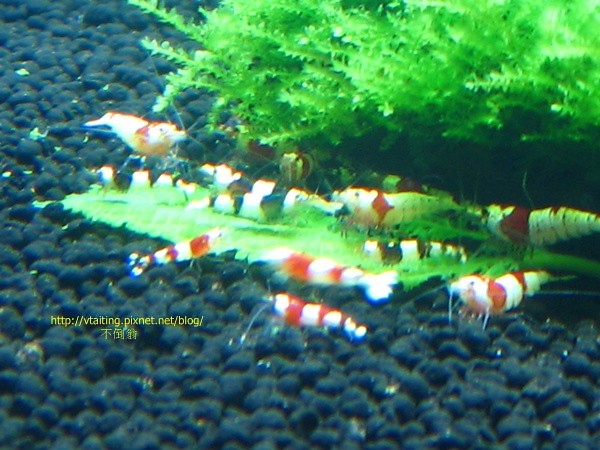The image depicts an array of red and white banded krill, resembling small lobsters, crawling on a green leaf or underwater plant that stands out against a dark background, possibly black stones underwater. Surrounding this scene is an abundant green, likely a bush or seaweed. The krill are clustered in the middle of the image, displaying their distinctive long whiskers and primarily red and white or white and black striped bodies. The overall scene suggests an underwater environment where these small crustaceans are feeding and moving around, perhaps in a natural underwater habitat rich with plant life.